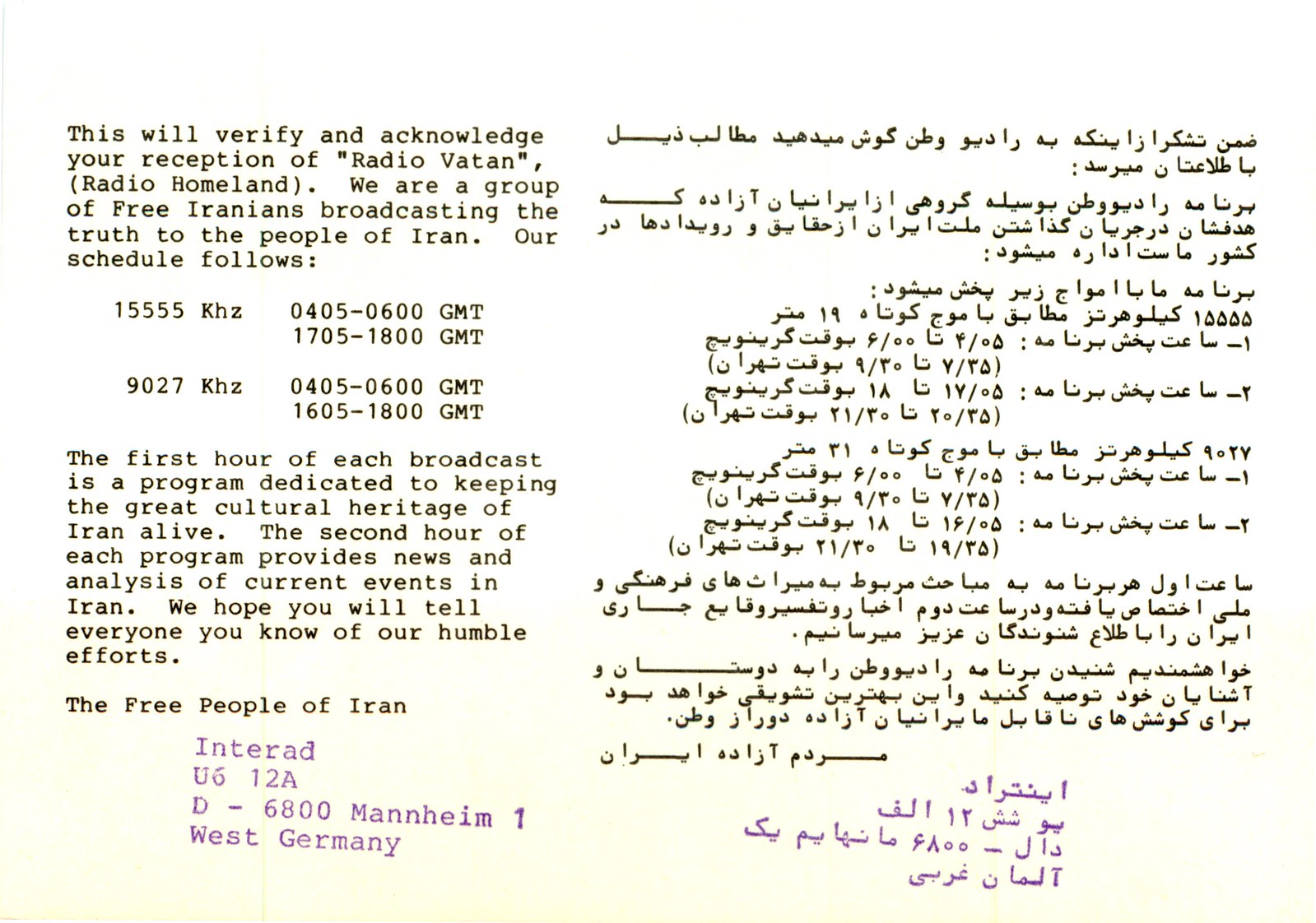The image is a detailed postcard intended to acknowledge the reception of Radio Vatan, also known as Radio Homeland, which is a broadcast from a group of free Iranians aimed at disseminating truth to the people of Iran. The postcard features text in both English and another language, possibly Persian, with the foreign text occupying the entire right side of the postcard. The English text is positioned on the left side, uniformly black except for a purple stamp at the bottom. It reads, "This will verify and acknowledge your reception of Radio Vatan, Radio Homeland. We are a group of free Iranians broadcasting the truth to the people of Iran. Our schedule follows." The text then details the broadcast schedule, with the first hour focusing on preserving Iran's cultural heritage and the second hour offering news and analysis of current events in Iran. The message concludes with a plea to share their efforts and is signed off by "the free people of Iran." At the bottom of the English section, the purple stamp notes "Interrad U612A D-6800 Mannheim, West Germany." The postcard's color scheme includes white, black, tan, and purple, emphasizing its official and poignant nature.